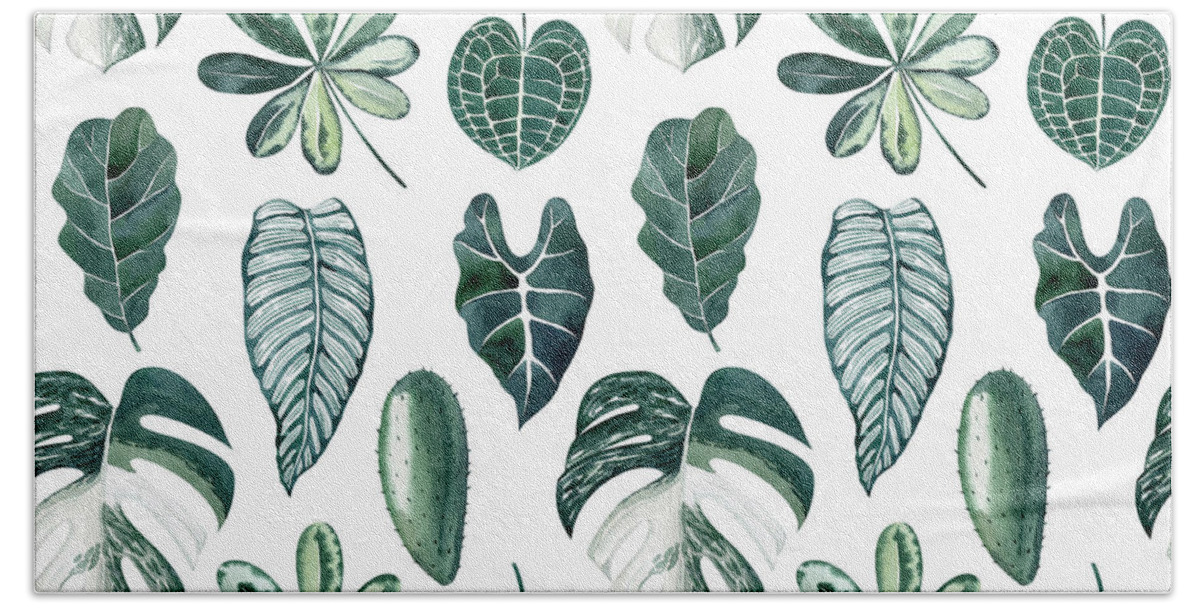This image showcases a stunning collection of tropical leaf patterns against a light gray background, creating a monochromatic palette predominantly featuring shades of green, white, and gray. The leaves exhibit a variety of shapes and designs, including pointed tips, heart-shaped leaves with intricate veining, and unnamed tropical leaves that evoke a daisy wheel appearance. Some leaves also display a unique two-tone coloration, with green and white segments, and a seashell-like leaf with white hairs prominently featured on the lower left and right corners. These exotic prints are highly versatile and are utilized on numerous surfaces, such as tablecloths, wallpaper, placemats, and even computer wallpapers. The overall pattern is a harmonious blend of natural elegance and artistic detail, ensuring it is both captivating and versatile for various decorative applications.